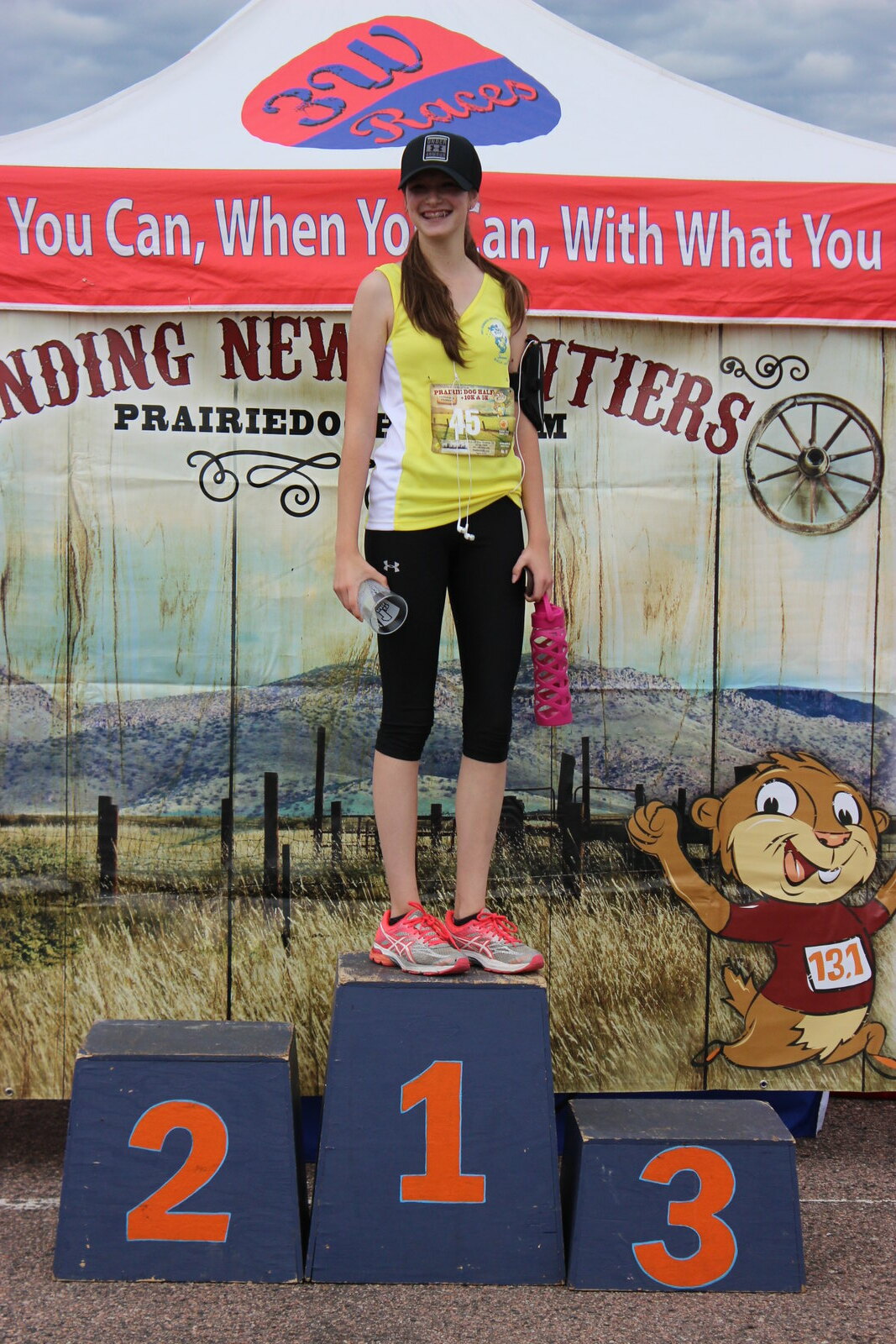In this outdoor image, a young woman stands proudly on the first-place podium of a race event. The blue podium with red numbers shows the placements one, two, and three, but she is the only person on the platforms. Dressed in athletic attire including a yellow tank top, black leggings, gym shoes, and a black baseball cap, she holds a trophy in one hand and a water bottle and phone in the other. Behind her is a large banner with the name "3W Races" prominently displayed in blue letters on a red background, and partially obscured encouraging statements like "You Can Win" and "Finding New Frontiers." A cartoon beaver dressed as a runner with the number 137 adds a whimsical touch to the banner. The setting appears to be a field or prairie, as suggested by the painted scene featuring tall grass and a wooden fence. The overall ambiance is celebratory and energetic.